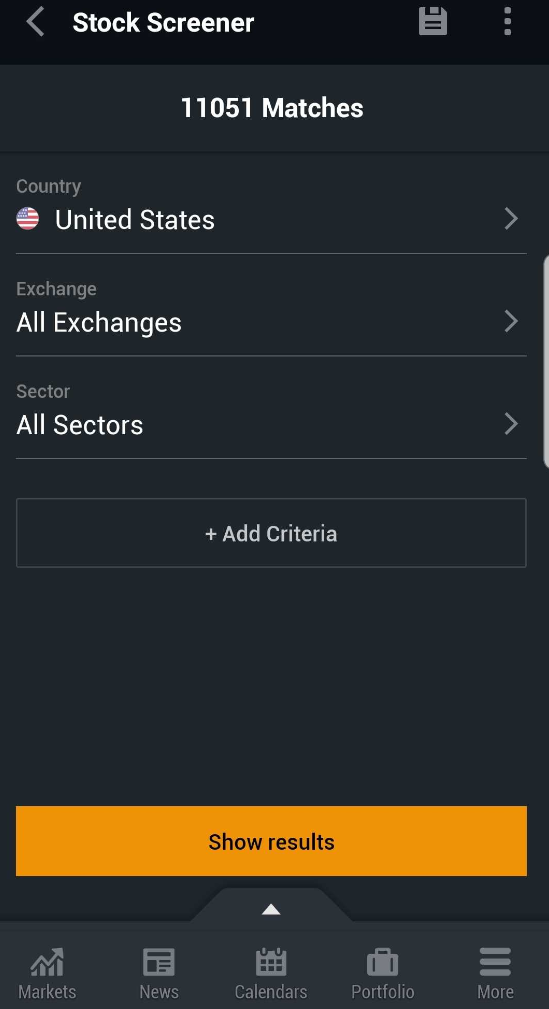The image is a screenshot from a cell phone app with a predominantly black background. On the right side of the screen, three horizontal dots are visible, possibly indicating a menu or additional options. 

Dominating the right side is a partially visible icon resembling a notebook, with the words "Stock Screener" prominently displayed in bold white letters. An arrow pointing to the left initiates the header.

Centrally located in bold white text is "11,051 matches," signifying the total number of results found. Underneath this, there is a filter section with various criteria:
- **Country:** Displaying the United States, indicated with a partial profile image of the U.S. flag and an arrow pointing right.
- **Exchange:** Showing "All Exchanges" in white, followed by an arrow pointing right.
- **Sector:** Indicating "All Sectors," also accompanied by a rightward arrow.

Below these filters is a white box with the text "Add Criteria" next to a plus sign, likely for adding more filters to refine the search results.

At the bottom of the screen is a large, prominent orange button stretching across the width of the screen with "Show Results" written in bold text. Directly beneath this button lies a navigation bar featuring icons for different sections of the app: Markets, News, and Calendars. The Calendars icon is highlighted, shown through an upward arrow extending from it. Adjacent to these icons are the "Portfolio" icon and a "More" option with three horizontal lines.

This detailed annotation captures all elements and functionalities as depicted on the mobile app screen.